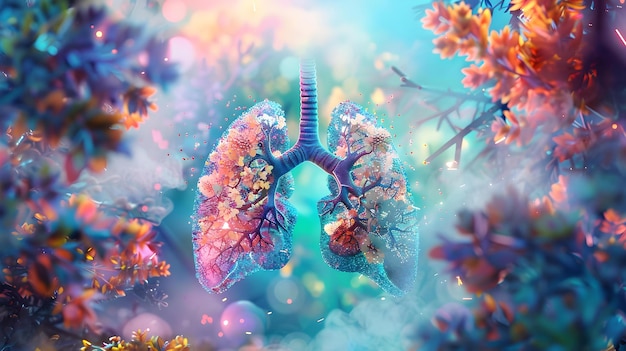The image showcases a stunning, whimsical representation of human lungs, set against a bright blue, sunlit sky. Suspended in mid-air, the lungs are intricately detailed, displaying a network of veins and airways that resemble the branches of a tree adorned with an array of flowers. These flowers, ranging in pastel and vibrant shades of pink, white, and hints of red, seamlessly integrate with the floral interior of the lungs, creating a harmonious color scheme. Surrounding the suspended lungs are flowering bushes and tree leaves in vivid hues of orange, blue, and purple. The background features a mix of slightly blurred foliage and confetti-like elements, enhancing the vibrant and enchanting quality of the image. Overall, the scene is a captivating blend of anatomical precision and artistic beauty, illuminated by the bright daylight.